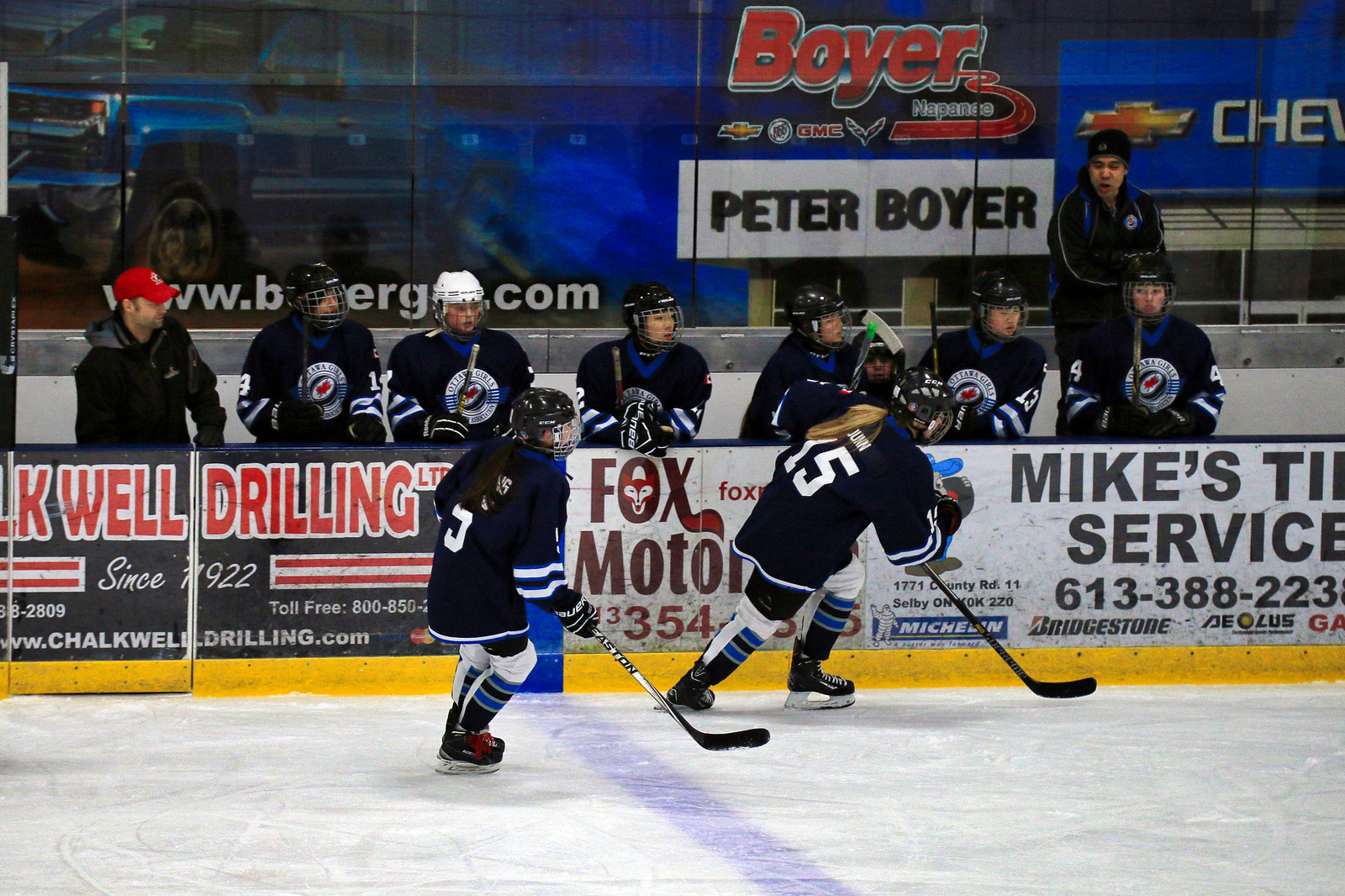The image captures a dynamic scene of a hockey game, focusing on the ice rink and the surrounding environment. On the rink, there are two female hockey players in action, both wearing black uniforms and helmets, skating towards the right with their hockey sticks poised. Behind them stands a row of teammates clad in the same black jerseys, leaning against the rink's barrier and attentively watching the game, hockey sticks in hand. Among the team members are two male coaches; one wears a red hat, and the other a beanie. 

The boundary of the rink is lined with advertisements, including "Well Drilling Limited," "Fox Motors," "Mike’s Tire Service," and "Boyer, Peter Boyer, Chevrolet." The clear plastic barrier above the advertisements reflects parts of these signs, creating a mirrored effect that shows the Chevrolet logo and a partial word "CHEV." To the left in the distance, there is a sign featuring a blue section with the Chevrolet logo and a vague image of a truck, indicating it's part of a larger ad. The overall scene is rich in detail, evoking the excitement and atmosphere of a live hockey match.